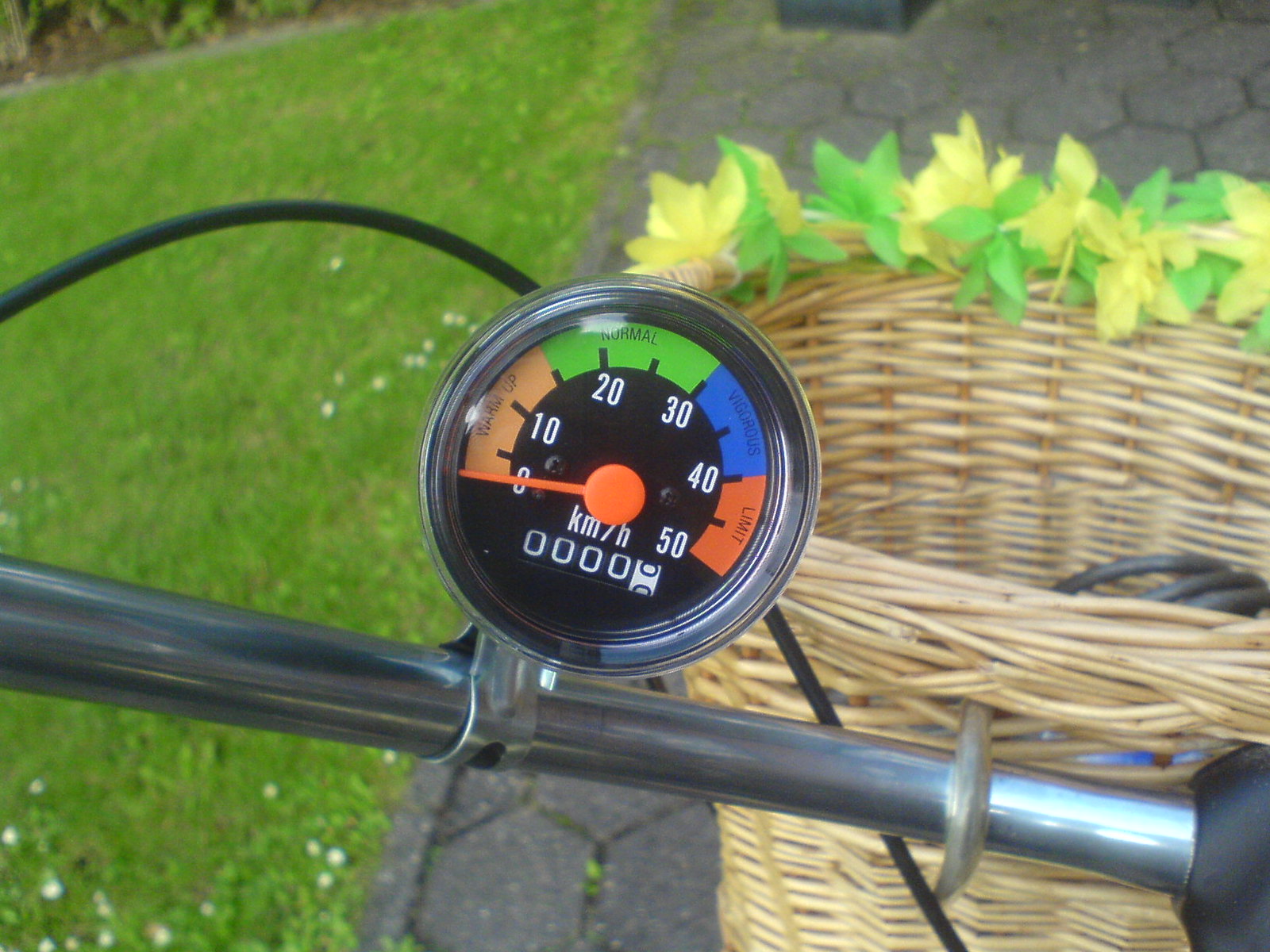A close-up image showcases the handlebar of a bicycle, illuminated brightly under natural light. The chrome handlebar glistens, adorned with a speedometer marked in kilometers per hour, ranging from 0 to 50. Color indicators on the speedometer signify various activity levels: orange for warm-up, green for normal, blue for vigorous, and red for limits. Attached to the front of the bicycle is a round, deep woven cane basket, intricately decorated with vibrant green and yellow flowers along its edge. Inside the basket lies a black, cord-like item, suggesting preparation for an outdoor journey. The background reveals a verdant lawn and a paved road, adding to the lively and inviting atmosphere of the scene.